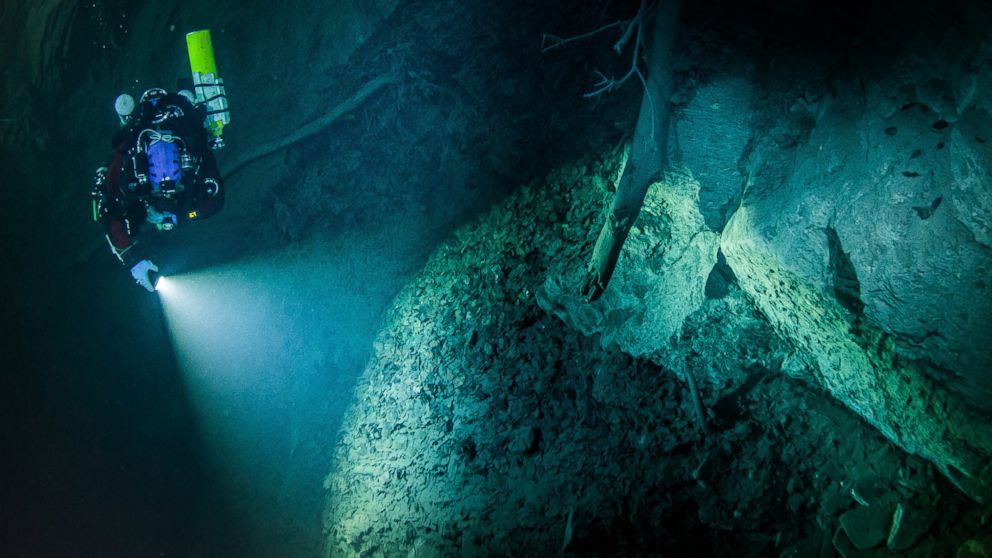In this detailed underwater photograph, a scuba diver clad in a black and reddish dive suit is captured from an aerial perspective. He wears a blue helmet and carries a bright yellow oxygen tank on his back. The diver, located in the top left of the image, is approximately 7 feet away from the camera. With his right hand, he shines a very bright flashlight on the rugged, greenish-hued rock formations that dominate the scene. The murky water necessitates the use of the flashlight, which distinctly illuminates a boulder on the right side of the image. A branch or tree formation extends upwards from the left side of this boulder, adding to the mystique. The overall environment suggests an underwater cave, devoid of fish or coral, with the rocky terrain and sparse vegetation setting a serene but mysterious backdrop.